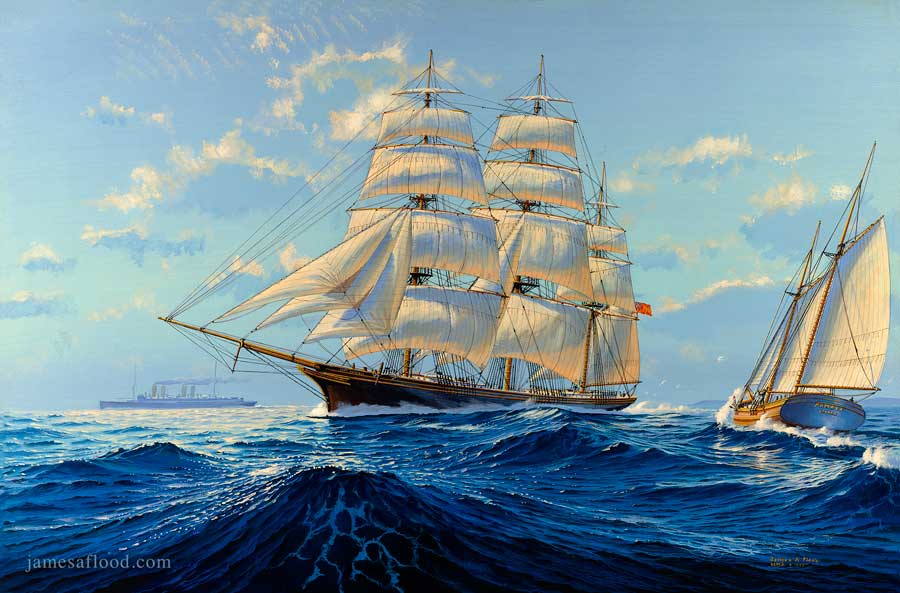In the painting by James A. Flood, prominently marked with "jamesaflood.com" in the bottom left corner, a dramatic maritime scene unfolds under a vibrant blue sky dotted with white clouds. The foreground features a sprawling ocean with choppy, tumultuous waves, likely stirred by wind or weather. Dominating this lively seascape is a majestic, brown sailboat with a multitude of sails—fourteen in total, distributed across its several masts. A striking red flag flutters at its stern. Slightly to the right, a smaller sailboat with just two sails appears to be making its way towards the larger vessel. On the distant left horizon, a grand steamship, reminiscent of the Titanic with smoke billowing from its smokestack, cruises calmly, adding historical gravitas to the scene. The painting skillfully balances the dynamic waves in the foreground with the three distinctively different boats, presenting a vivid narrative of nautical adventure.